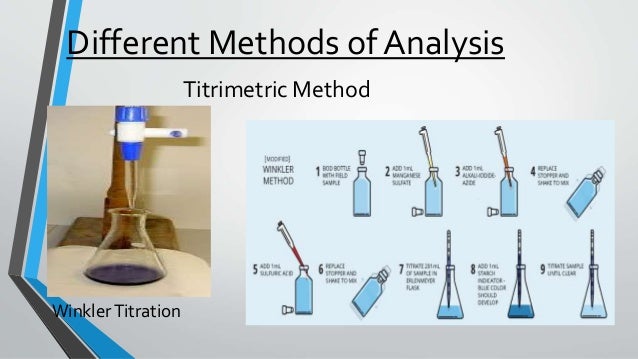The image is a detailed visual guide for the Winkler Titration method, a specific type of titrimetric analysis. The background is a light blue, with a gray and bright blue stripe running down the left side. At the top, in bold, underlined black text, it reads "Different methods of analysis." Below this title, the phrase "titrometric method" is displayed in a slightly smaller font.

On the left side of the image, there is a real photograph showing the Winkler titration in action. It features a beaker with a small amount of blue liquid at its bottom, and a blue-topped dropper positioned above, with liquid dripping into the beaker.

The right side of the image consists of a step-by-step diagram illustrating the nine steps of the Winkler method. The steps involve various actions such as removing and replacing a bottle cap and using a syringe or eyedropper to handle liquids. Each step is numbered and accompanied by a small illustration, guiding the viewer through the entire titration process. The subtitle "Winkler Titration" appears in black lettering at the bottom left of the diagram.